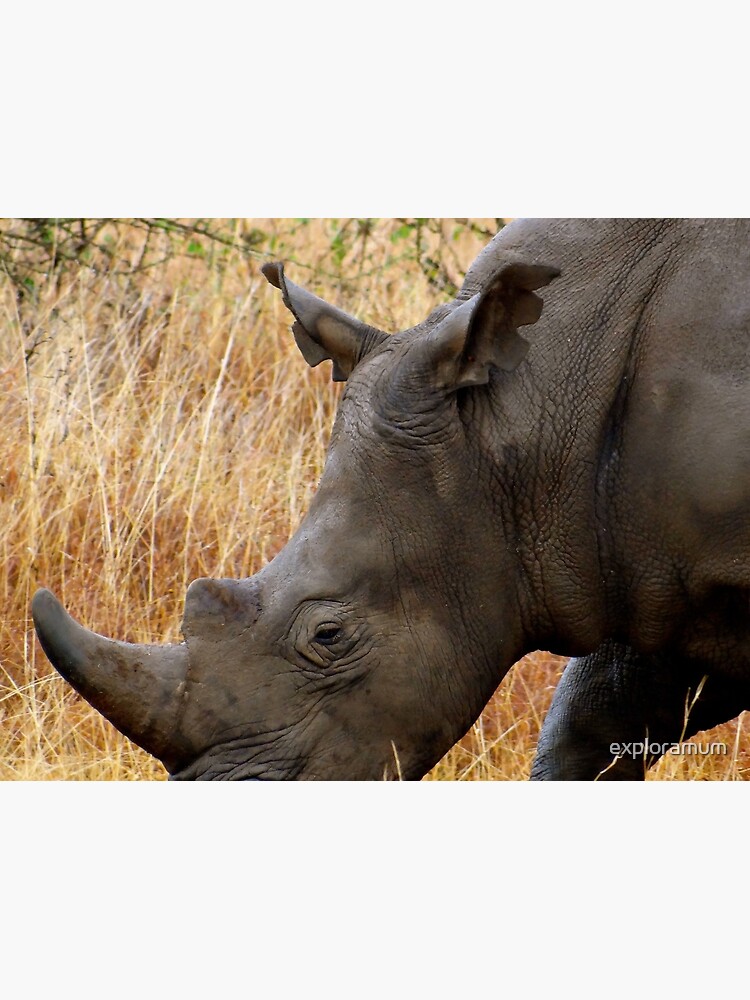This is a detailed photograph of a rhinoceros focusing mostly on its head, upper body, and part of one front leg. The rhino, characterized by its gray, wrinkled skin, is facing to the left, allowing a clear view of its larger front horn and a smaller horn positioned further back. Its visible eye and two ears add to the expression captured in the image. The background consists of a tan and orange straw or hay, giving an earthy tone to the setting. In the upper left corner, black tree branches with green leaves are visible, while the bottom right corner features the word "Explorium" written in light gray, transparent text.